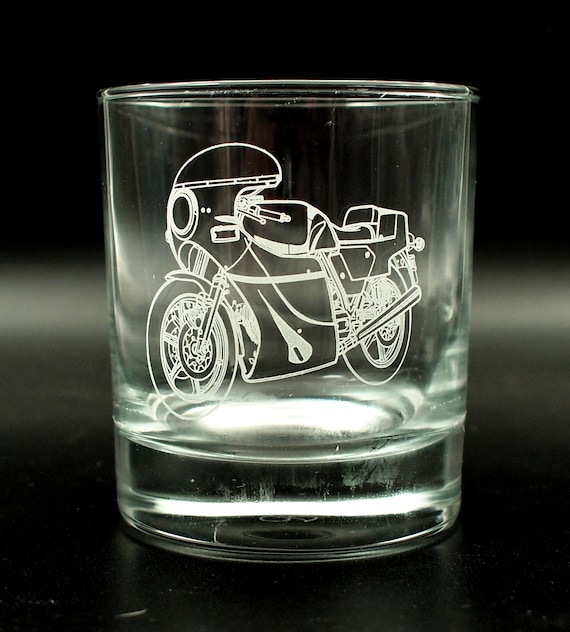The image features a highly detailed, close-up view of a clear, glass cup set against a predominantly black background with some blurry gradients of dark and light gray. The cup is short with a thick glass base and a small rim. Adorning the front of the cup is an intricate white sketch of a sports motorcycle. This detailed etching showcases thin wheels, a large exhaust pipe over the rear wheel, and a long seat with a small storage canopy at the back. The motorcycle's design includes a short windshield, large headlight at the center front, and visible handlebars extending to the right. The photograph is well-lit, highlighting the clear quality of the glass and the distinctness of the precise motorcycle sketch. The intense zoom of the image ensures that the focus remains entirely on the glass cup and its detailed artwork.